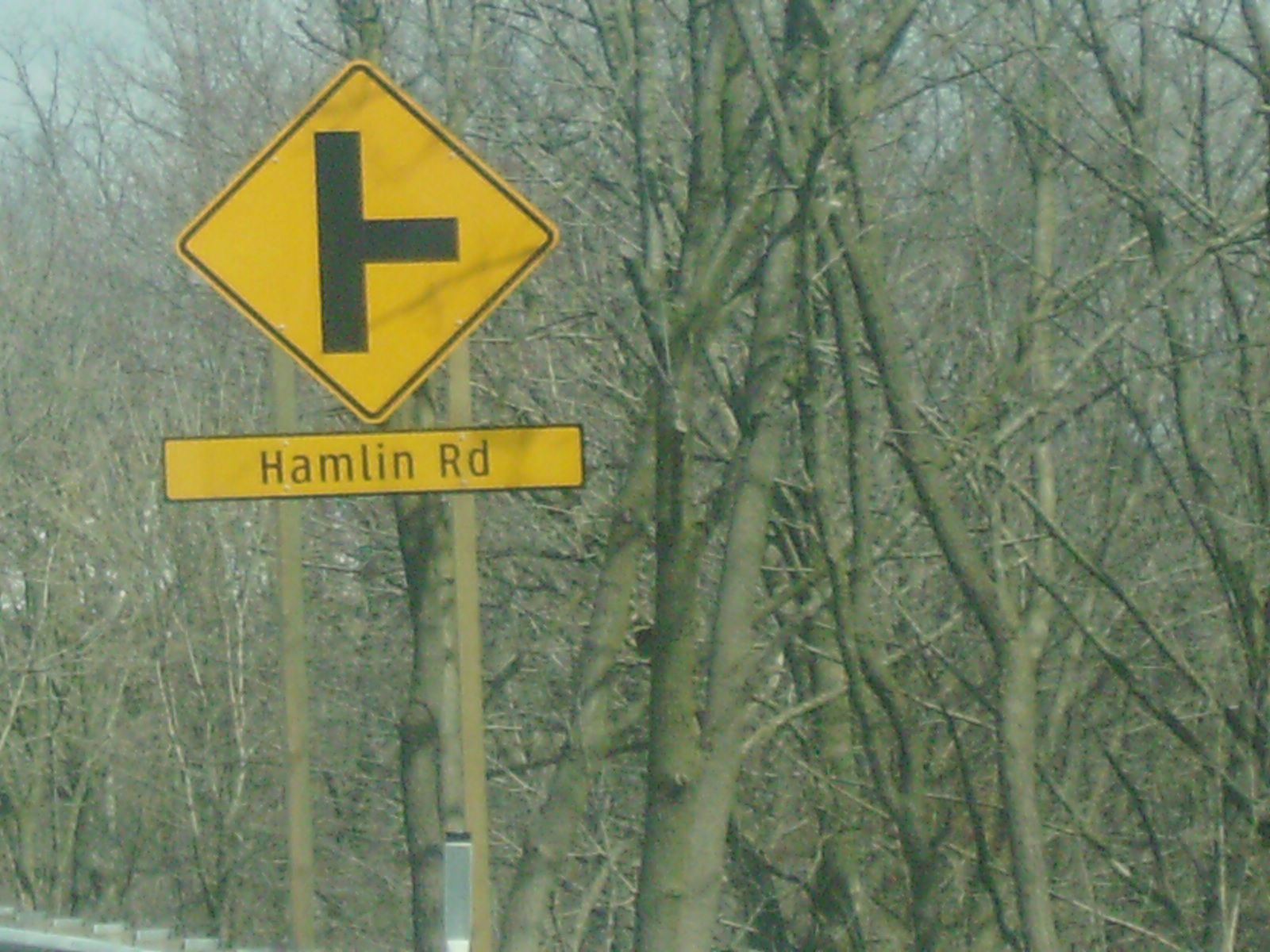This photograph captures a roadside scene in a wooded area, likely taken during late autumn or winter, as most of the trees in the background are bare of foliage. Central to the image is a bright yellow diamond-shaped road sign with a thin black border. The sign features a rotated T-shaped symbol, with the middle part pointing right and the vertical line extending up and down. Below this is a rectangular yellow sign with the text "Hamlin Rd." Both signs are mounted on a wooden post, secured with screws—four on the upper sign and two pairs on the lower sign. At the bottom left corner of the image, a guardrail is partially visible, suggesting the road may curve or be elevated, such as on a bridge. The sky in the background is a grayish-blue, lending a muted tone to the overall scene.